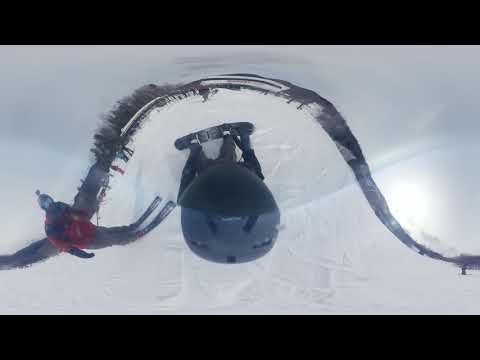This image appears to be taken on a ski hill or snowy mountain using a GoPro or similar action camera, providing a distorted, fisheye perspective. Centrally, it features the black helmet of a snowboarder viewed from an aerial angle, creating a dark, arch-like shape in the center of the image. The helmet has noticeable indents, likely designed for ventilation. To the left of the snowboarder, a skier dressed in a red jacket and equipped with goggles and a GoPro on their helmet is visible. The snowy background appears wavy due to the camera's rounded lens effect, and other figures can be seen in the distance, enhancing the sense of depth and creating the illusion of a hill weaving across the scene. The image is bordered by a dark frame at the top and bottom, measuring approximately five by four inches.